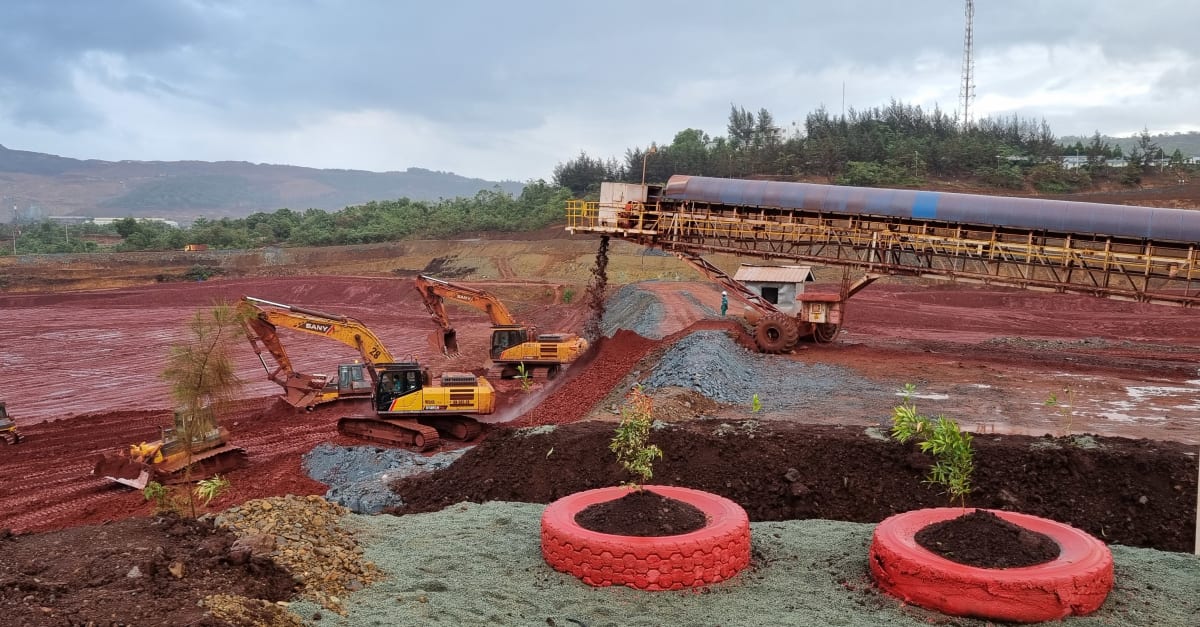This photograph captures an eye-level view of an early-stage construction site beneath a cloudy, grayish sky. The background features rolling hills to the left, dotted with green and brown patches, while to the right, a towering radio antenna stretches out of the frame. Closer to the photographer, a line of bushes and smaller trees marks the horizon. Dominating the foreground is a deep, reddish-brown expanse of freshly dug earth, interspersed with large construction machinery, including two diggers on the left and two bulldozers—one driving and another positioned leftwards. On the right, a prominent conveyor belt is seen transporting this earth from higher ground into a depression below. A small figure can be discerned in the distance, amidst the operation. Near the bottom of the photo, closer to the photographer, two spray-painted pink tires house two small trees each, with an additional little pine tree planted directly into the dirt.